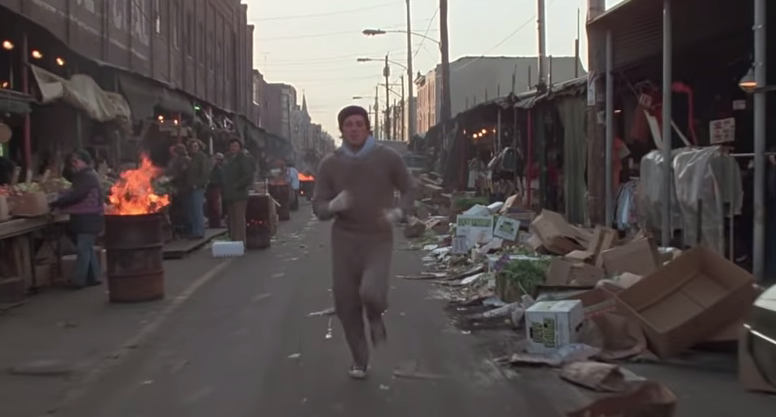The image is a semi-blurred digital photograph, likely a screenshot from the classic movie "Rocky." It captures a moment where Rocky is running through a gritty, downtown district during his morning exercise. He is dressed in his iconic gray sweatpants and a hat, jogging down the middle of a street lined with buildings that stand about two stories tall. The scene is set during the daytime, under a clear but somewhat murky sky.

To the left of Rocky, a series of small market shops are visible, where people are busy selling fruits, vegetables, and clothes displayed on portable roll-away hangers. There are metal barrels lit with fire, suggesting a cold day, and providing warmth to the vendors and shoppers. On the right side, the street is cluttered with piles of trash and empty cardboard boxes, emphasizing the impoverished area’s bleakness.

The colors in the image are predominantly gray and brown, with sporadic hints of green, white, black, and the yellow-orange glow of the fire barrels. The street stretches out towards the horizon, with more buildings and streetlights in the background, further enhancing the downtown setting.